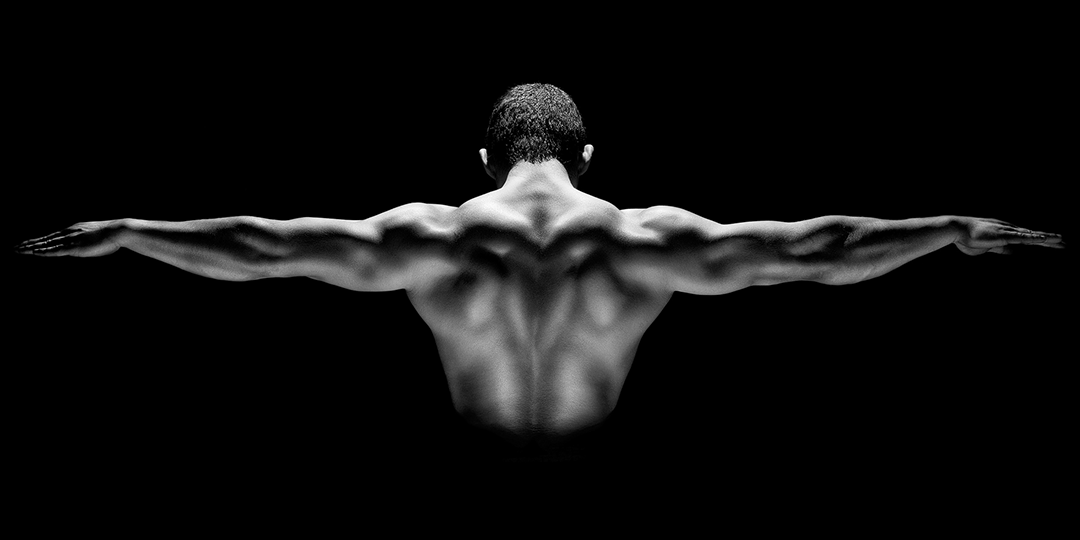This black and white art photograph captures the muscular back of a man, viewed from the waist up with a completely black background. He stands shirtless, arms fully outstretched like wings, showcasing an extensive wingspan. His head is slightly bowed, accentuating the definition in his triceps, biceps, deltoids, and overall back musculature. The dramatic lighting from above and below highlights his physique, casting shadows that enhance the contours of his muscles. His short, dark hair and ears are visible, hinting at his possibly African American heritage, though the monochromatic tones render exact details ambiguous. The photograph is a striking portrayal of masculine strength and the aesthetic beauty of the human body, emphasizing the artistic and slightly erotic essence of the image.